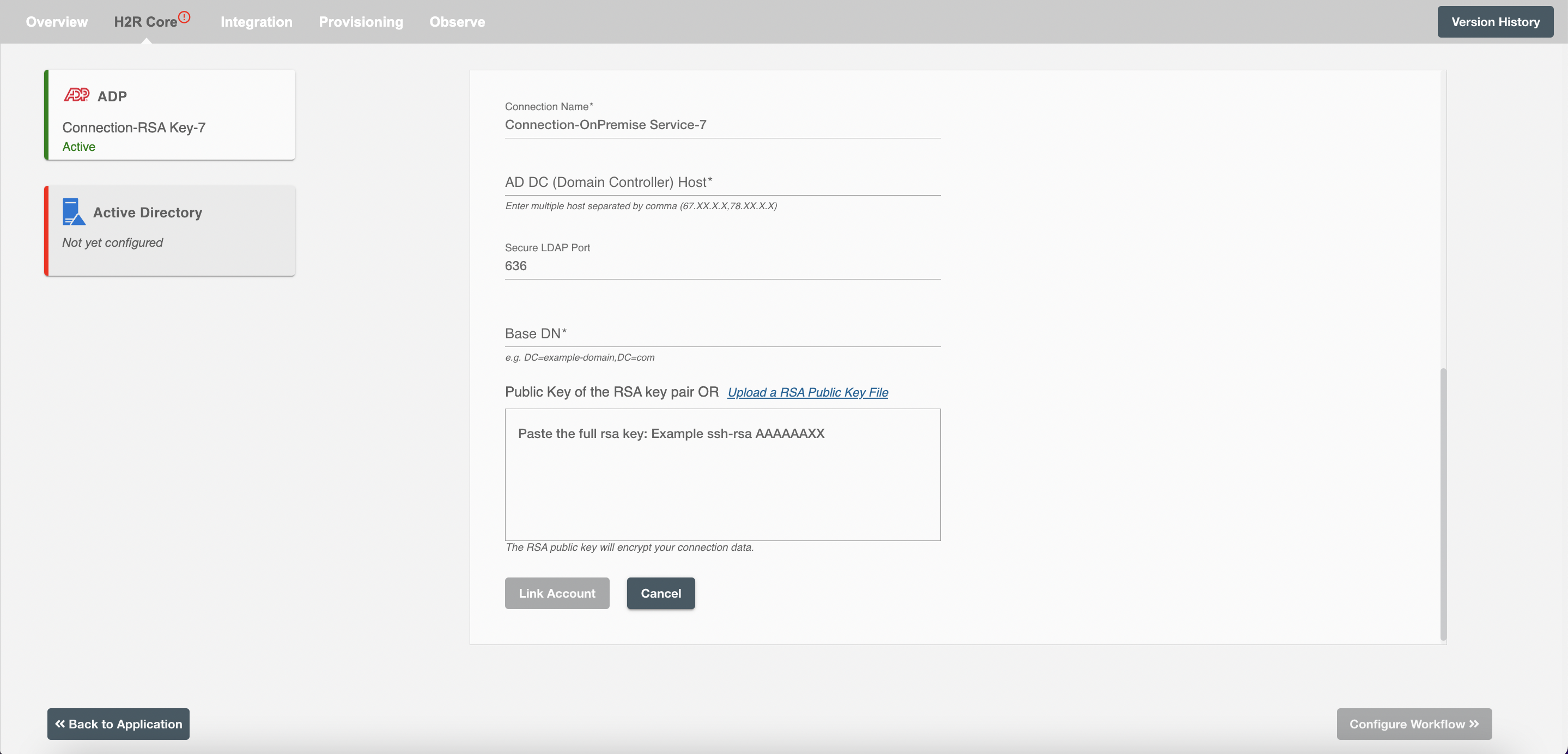This is a detailed screenshot of a web page, showcasing a user interface for managing H2R Core integrations. 

At the top, a gray navigation bar spans the width of the page. From left to right, it features the following sections: "Overview" in white lettering, "H2R Core" in black lettering, and additional tabs labeled "Integration," "Provisioning," and "Observe." On the far right of this bar, there is a prominent black button with white lettering that reads "Version History."

Below the navigation bar, the "H2R Core" tab is highlighted. The content area below this selection displays two sections. The first section, outlined in a square, is titled "ADP Connection" and indicates an RSA Key 7 status as "Active." The second section, also outlined in a square, is labeled "Active Directory" but is marked as "Not Yet Configured." 

At the bottom of this content area, there is a link labeled "Back to Application."

On the right-hand side of the page, a form is displayed within a white square. This form includes several fields for input:

- **Connection Name**
- **Connection On-Premise Service 7**
- **ADDC Domain Controlled Host**
- **Secure LDAP Port 636**
- **Base DN**

Below these fields, there is an instructional section for RSA key configuration. It includes a placeholder box labeled "Paste the Full RSA Key Example SSH-RSA-AAAAAAAXX." An adjacent clickable link, displayed in blue and underlined, reads "Upload a RSA Public Key File." 

Further down, the form mentions, "The RSA Public Key will be encrypted for your connection data," providing reassurance about security. At the bottom of this form are two buttons: a gray "Link Account" button and a black "Cancel" button.